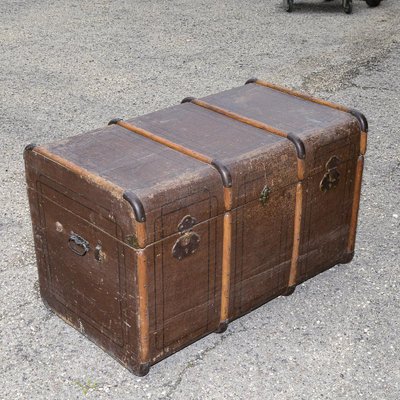The image depicts an old, worn-out wooden chest resting on a cracked and stained gray concrete ground. The chest, which appears to date back to the 1920s or 1930s, has a faded whitish lid that reveals its original dark brown color along the sides and front. Positioned diagonally, the chest's front end points towards the lower left corner of the picture, while the back end faces the upper right. The chest features three clasps on the front, a handle on the left side, and darker brown protective corners. The concrete surface beneath it shows various cracks and stains, with an indistinguishable gray and black object faintly visible at the top of the image.